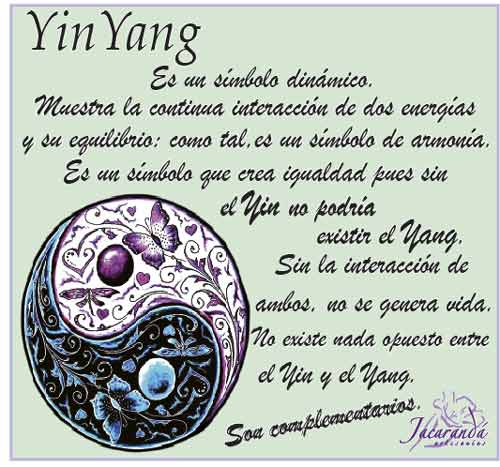The image features an intricately detailed depiction of a Yin Yang symbol, centered on a light green background. The Yin Yang symbol is divided into two halves: the top half is adorned with lighter purple, white, and green hues, and festooned with butterflies, hearts, flowers, and swirling patterns. The bottom half showcases shades of blue and black, similarly adorned with flowers, butterflies, and hearts. A black border circle on the left bottom, resembling a peace sign, adds an additional element to the composition.

At the top of the image, the text "Yin Yang" is prominently displayed, rendered in an ornate script that appears to be in a different language, possibly Spanish, describing or providing the history of Yin Yang. This text cascades from the middle, extending downwards, filling much of the page with its elegant script. On the bottom right-hand side, there is a logo or artist’s signature that reads "Jacqueline Navina." The confluence of colors – black, green, gray, pink, purple, and blue – along with the stylized writing, merge to create a visually appealing and richly symbolic image that could easily belong in an article or a book.